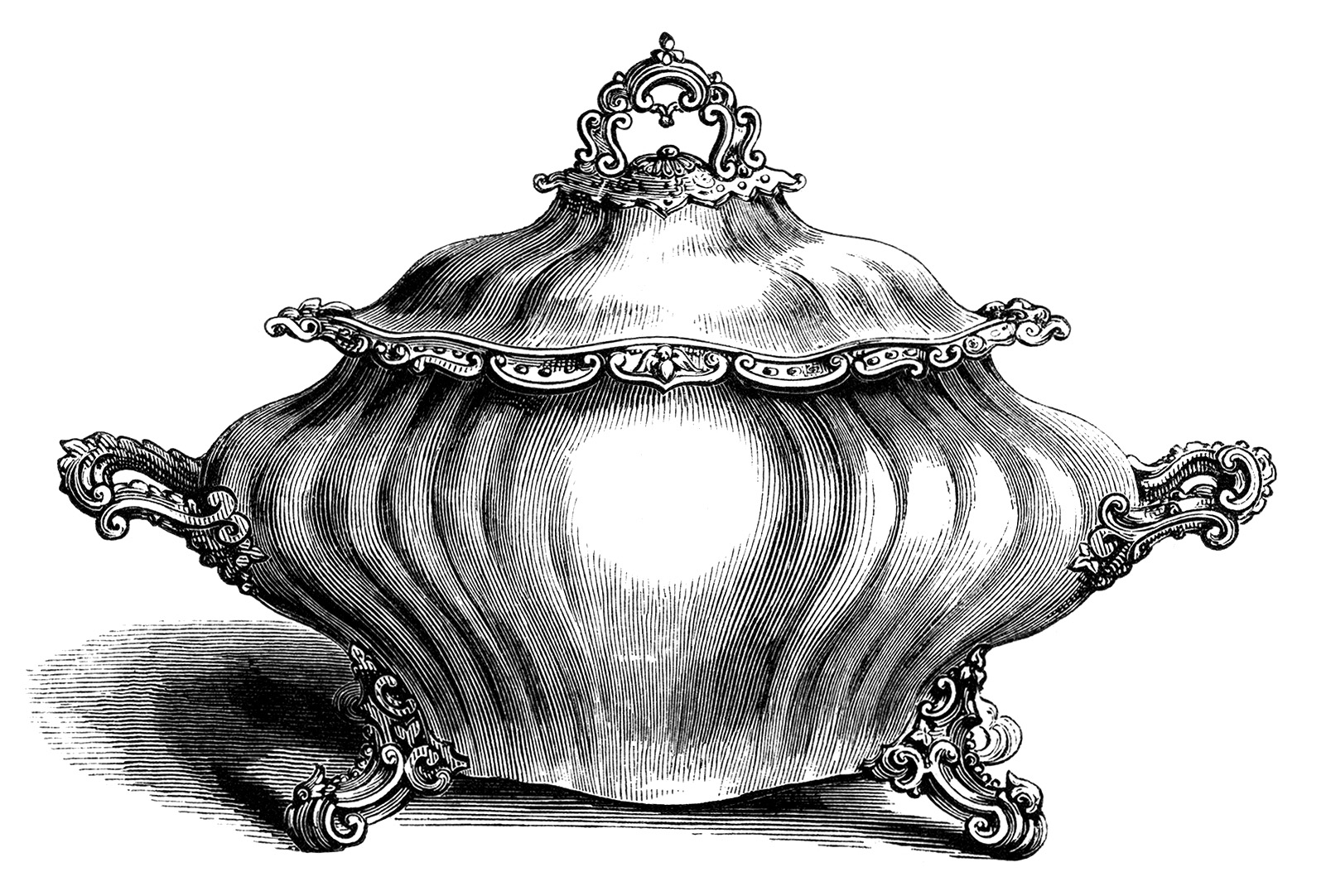This black and white artistic drawing depicts an ornate, antique-like container resembling a vase or a silver gravy pot with a dome-shaped lid. The centerpiece of the container is stark white, seamlessly connecting to the intricately patterned handles and short, decorative legs that support it. The dome lid features an elaborate handle at the top, held in place by four S-shaped supports that form an arch, allowing for easy lifting. The sketch is carefully detailed with finely drawn lines in various shades of black and gray, adding depth and dimension to the ribbed surface of the vessel. The container casts a subtle shadow, suggesting a light source from the upper right. The entire image stands out against an entirely white background, devoid of any text or numbers, emphasizing the delicate craftsmanship of the drawing.